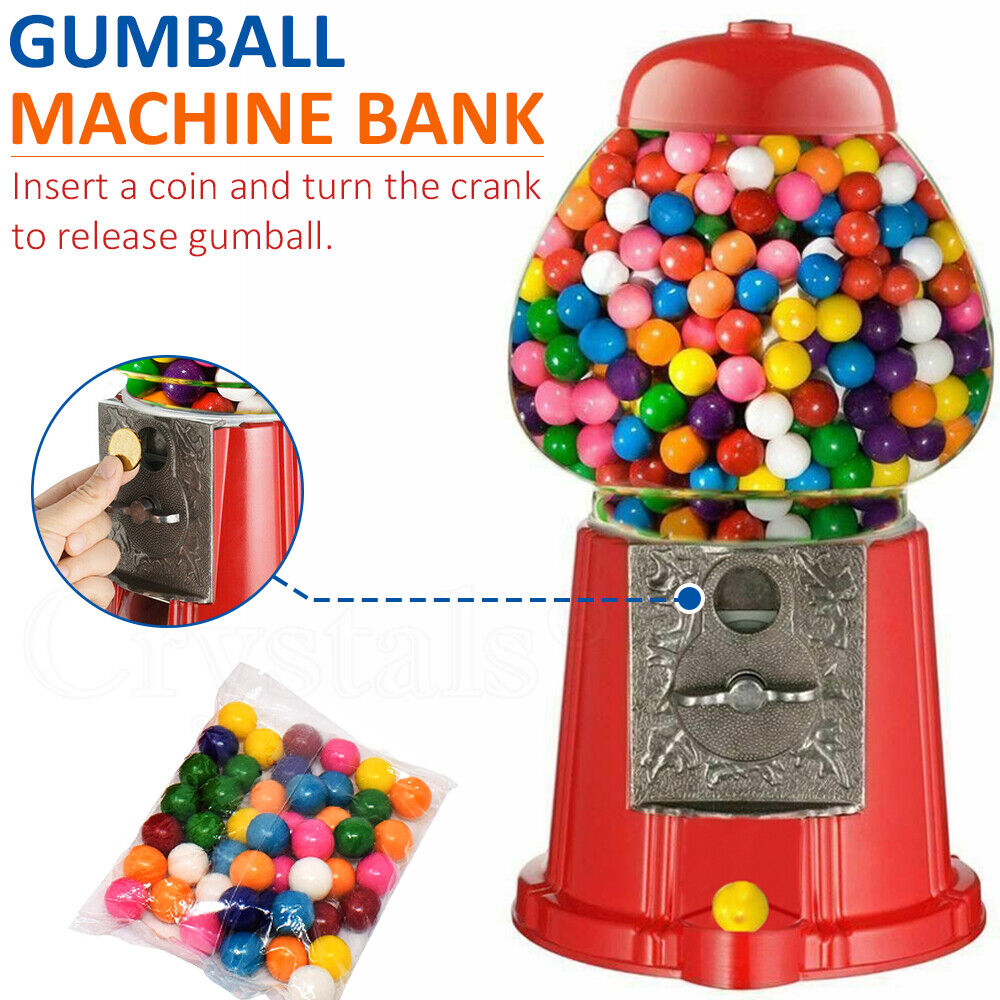This detailed image features an old-style gumball machine, showcasing a striking red base and a matching red metal cap atop a clear plastic or glass globe filled to the brim with colorful gumballs. The gumballs come in a spectrum of colors, including white, blue, yellow, orange, purple, red, green, and pink, contributing to a vibrant and eye-catching display.

In the upper left-hand corner, blue capitalized text reads "GUMBALL," followed by orange capitalized text declaring "MACHINE BANK." An orange underline accentuates this title, and directly beneath it, non-capitalized text with a capitalized first letter instructs, "Insert a coin and turn the crank to release a gumball." 

Below this text, a circular inset image effectively demonstrates the coin insertion process, showing a hand holding a gold coin poised to enter the metal coin slot of the gumball machine. Adjacent to this inset, the machine's mechanism is partially visible, with a yellow gumball ready to be dispensed.

Additionally, the advertisement includes a plastic pack filled with an assortment of gumballs, emphasizing the colorful variety available. The gumball machine's central section, featuring a sturdy gunmetal finish, highlights the coin slot and crank, while the lower part shows a yellow gumball being dispensed. This comprehensive depiction combines textual and visual elements to effectively convey the functionality and appeal of the gumball machine bank.